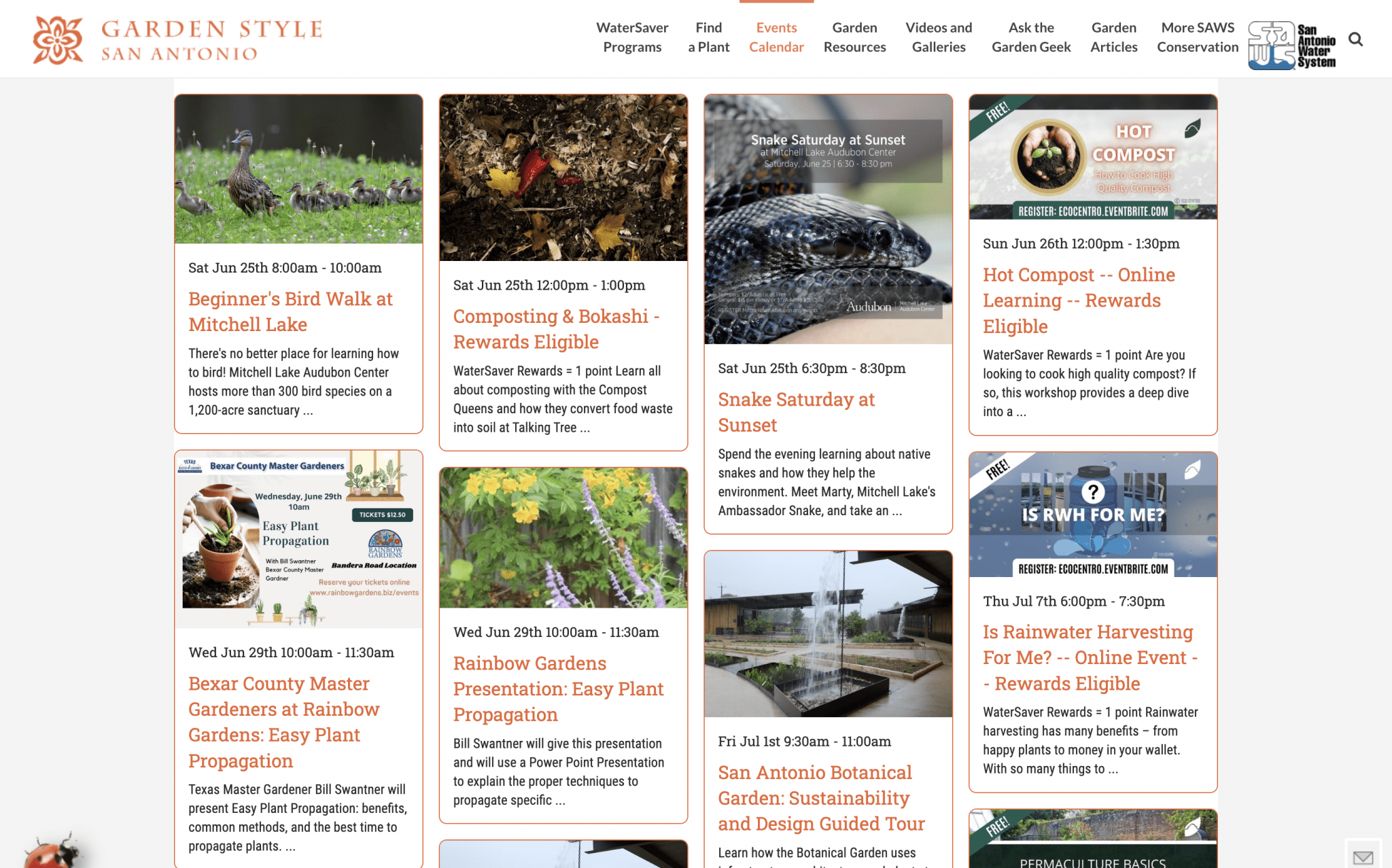In the top-left corner of the image, the phrase "Garden Style, San Antonio" appears in bold orange letters beside a delicate, orange-outlined flower illustration. To the right, there is a navigation menu with black text, listing: "Water Saver Programs," "Find a Plant," "Events Calendar" (highlighted with an orange underline), "Garden Resources," "Videos and Galleries," "Ask the Garden Geek," "Garden Articles," and "More SAWS Conservation." Nearby, the "San Antonio Water System" logo and a search bar are also present.

Below the menu is a detailed event schedule, meticulously organized and bordered with thin orange lines. The highlighted entries are:

1. **Saturday, June 25, 8:00 AM - 10:00 AM**  
   - In black: "Beginners Bird Walk at Mitchell Lake."

2. **Saturday, June 25, 12:00 PM - 10:00 PM**  
   - In orange: "Composting and Bokashi, Rewards Eligible."

3. **Saturday, June 25, 6:30 PM - 8:30 PM**  
   - In black: "Snake Saturday at Sunset," illustrated with black snake images.

4. **Saturday, June 26, 12:00 PM - 1:30 PM**  
   - In orange: "Hot Compost, Online Learning, Rewards Eligible."

5. **Wednesday, June 29, 10:00 AM - 11:30 AM**  
   - In orange: "Bexar County Master Gardeners at Rainbow Gardens, Easy Plant Propagation."

6. **Wednesday, June 29, 10:00 AM - 11:30 AM**  
   - In orange: "Rainbow Gardens Presentation, Easy Plant Propagation."

7. **Friday, July 1, 9:30 AM - 10:00 AM**  
   - In orange: "San Antonio Botanical Garden, Sustainability and Design Guided Tour."

8. **Thursday, July 7, 6:00 PM - 7:30 PM**  
   - In orange: "Rainwater Harvesting for Me... Online Event, Rewards Eligible."

At the very bottom, there are indications of two more cut-off advertisements or events.